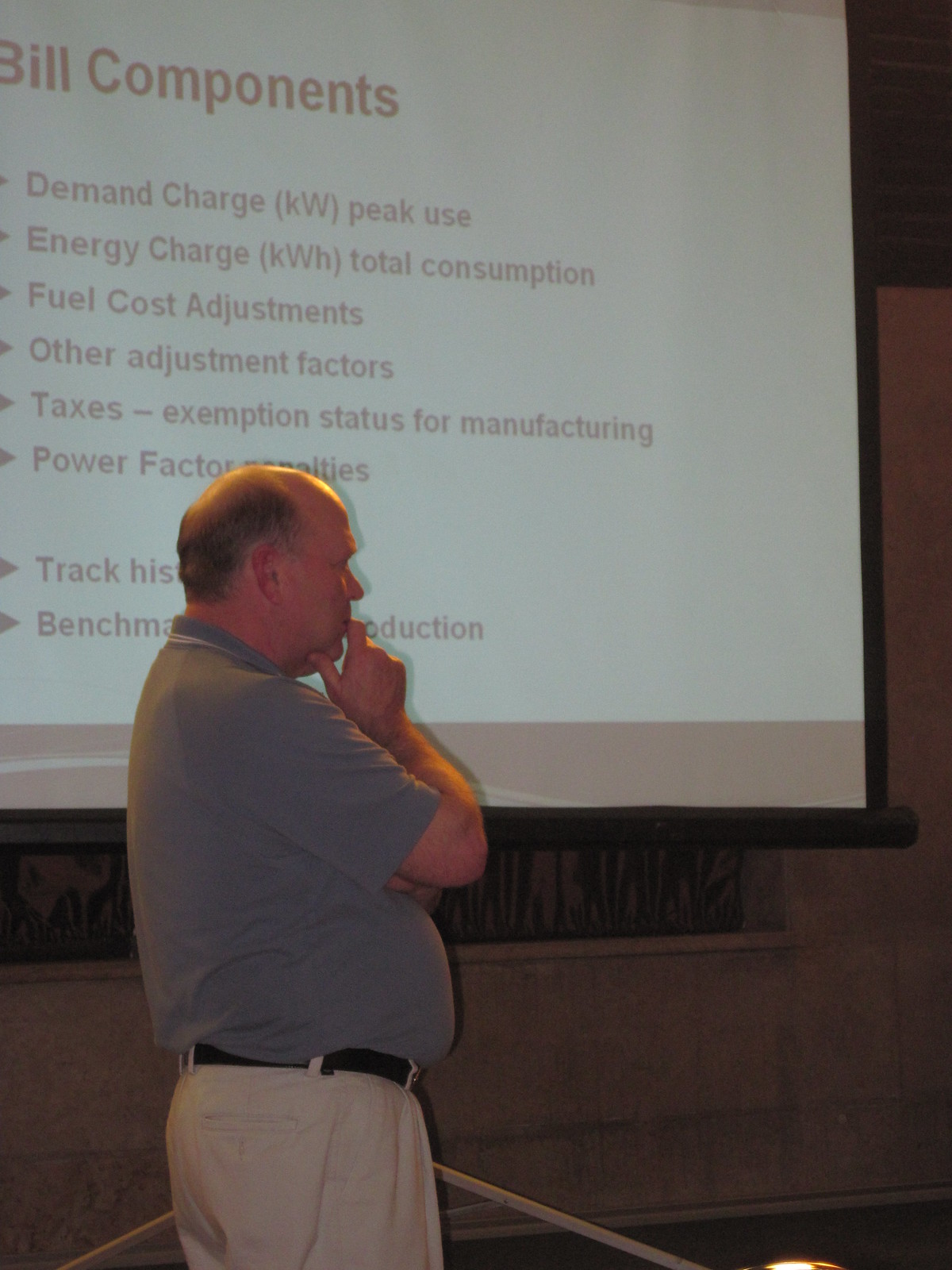This vertically aligned rectangular image captures a side view of a middle-aged man with a contemplative expression, positioned in the bottom left corner. He is slightly heavyset, dressed in a gray short sleeve polo shirt and khaki pants secured with a black belt. His balding head reveals short brown hair at the back and sides. His right hand is raised to his chin and mouth, suggesting he is deep in thought. Behind him is a large projected screen displaying a presentation with the bold black title "Bill Components." The screen features bullet points marked by right-pointing triangles, listing items such as "Demand Charge, KW Peak Use," "Energy Charge, KWH, Total Consumption," "Fuel Cost Adjustments," "Other Adjustment Factors," and "Taxes, Exemption Status for Manufacturing." Due to the man's partial coverage, some text is obscured, including "Power Factor Specialties." The presentation continues with additional hidden bullet points. This indoor scene suggests a conference or trade show setting where the man appears engrossed in the details of the projection. The predominant colors in the image are gray, tan, white, black, and hints of orange.